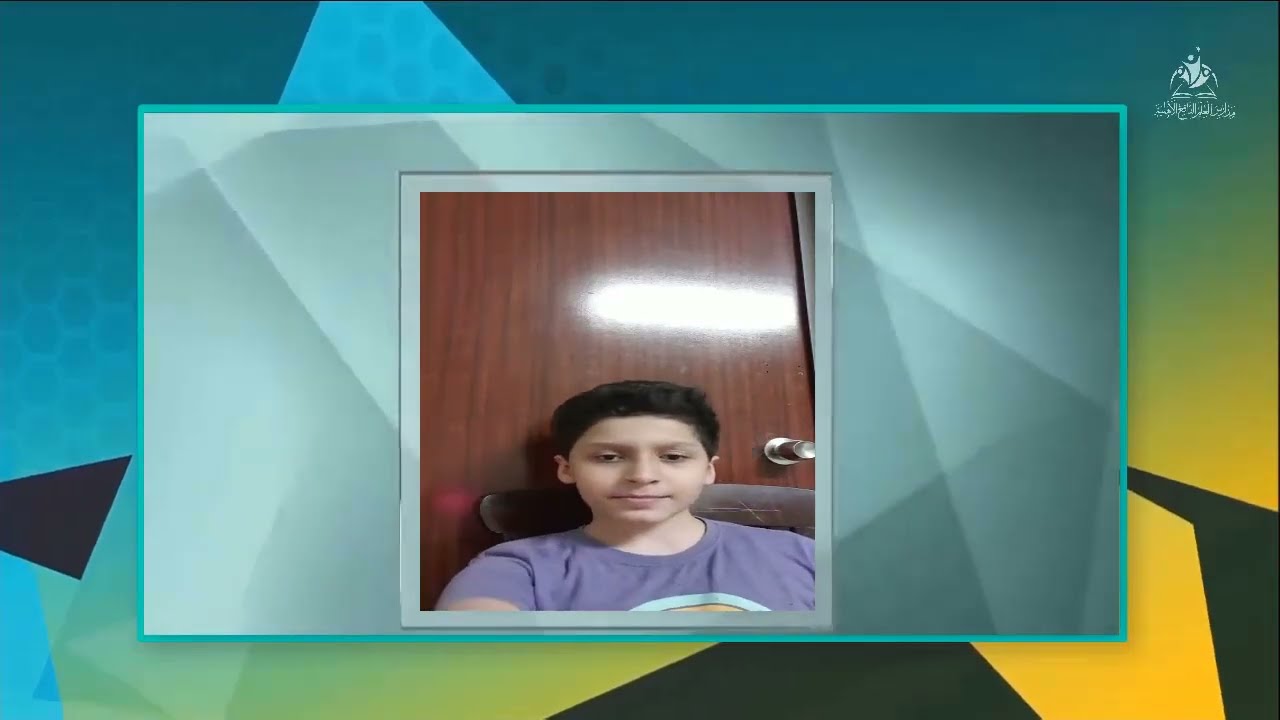The image is a multi-framed composition featuring a young boy. The outer frame showcases a vibrant, abstract art background with bright, deep turquoise hues adorned with darker round circles and honeycomb shapes. The background transitions from teal in the top left to yellow in the bottom right, interspersed with wonky triangular shapes at weird angles, some black but mostly blending in gradient colors. The top left corner features a logo of a person skipping alongside Arabic writing. The inner picture is bordered with a light turquoise frame and a gray backdrop composed of triangulated lines, lightening from right to left. Centrally, there is another white-framed portrait of a serious-looking boy, about 12 years old, with brown or black hair. He is seated in a brown chair in front of a dark wooden door with a silver handle and a light reflection in the middle. He wears a short-sleeved purple shirt, possibly with a logo. The overall image combines multiple layers and intricate details, blending vibrant and neutral colors with abstract and structured elements.